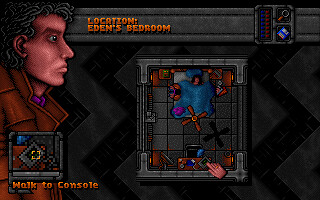The image is a still frame captured from a video game featuring an overhead view of a bedroom. The focal point is the profile portrait of a character cloaked in a brown trench coat with the collar stylishly popped. The room is meticulously detailed, showcasing a ceiling fan, a neatly made bed, a desk, end tables, and various other personal items that add to the realism of the scene. A text bar across the top of the screen reads "Location: Eden's Bedroom," accompanied by an icon of a magnifying glass, indicating that interactive elements may be present for exploration. At the bottom, a map is superimposed with the instruction "Walk to Console," guiding the player toward their next objective within the game.